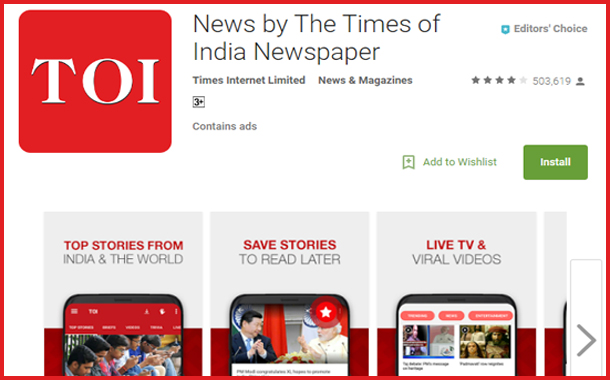The image from the Times of India (TOI) website displays a visually striking logo featuring three white letters within a red box with rounded edges. This logo is prominently placed inside a larger, white box outlined in red with a grayish print. The accompanying text reads "News by the Times of India Newspaper, Times Internet Limited, News and Magazines," indicating that the content is ad-supported and marked as the editor's choice.

Adjacent to this text is a blue icon, and the app has garnered a 4 out of 5-star rating from 503,619 users. There is an option to add the app to your wish list, and a green "Install" button with white lettering invites users to download the application.

Below this section, the caption "Top Stories from India and the World" introduces several images displayed on the tops of phones. One image shows Indian people who appear to be praying, with a feature allowing stories to be saved for later reading. Another image features the Pope engaging in conversation with another leader, under the heading "Live TV." There is also a section labeled "Viral Videos," showcasing two video thumbnails.

An arrow on the right indicates additional content available beyond the visible portion of the image, inviting users to explore more.